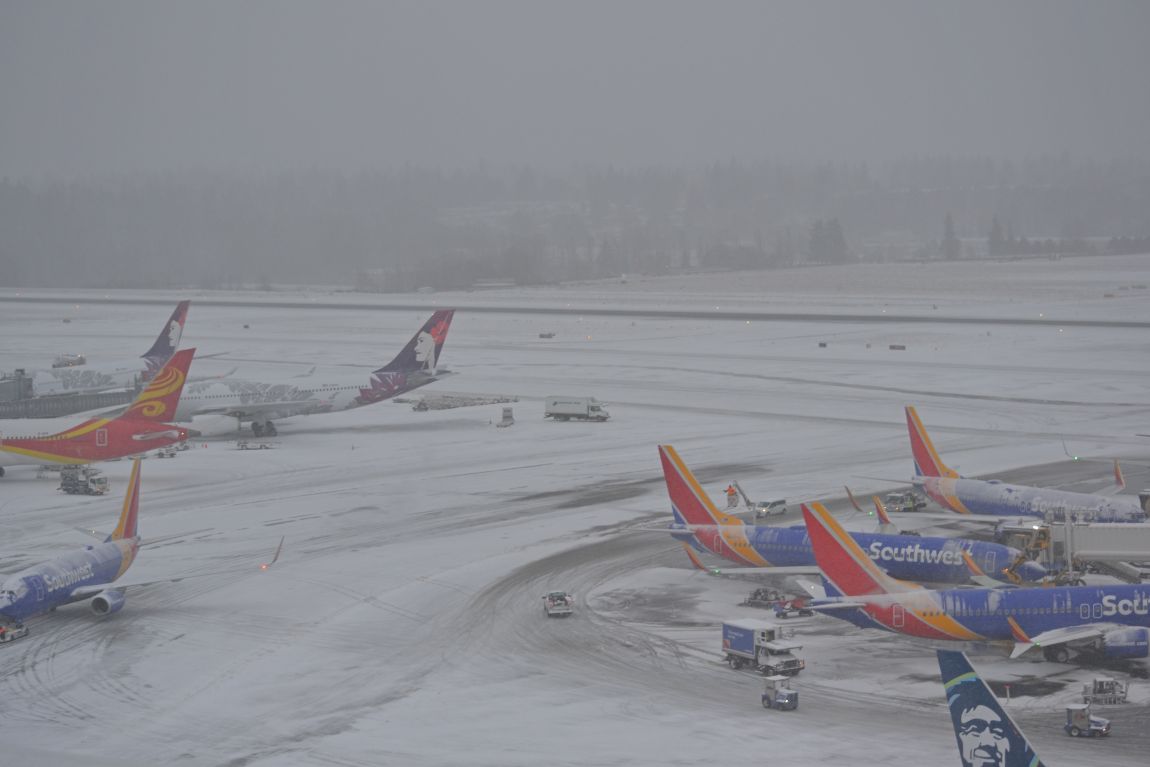This photograph captures an aerial view of a snowy airport tarmac bustling with activity. In the bottom right quadrant, three Southwest Airlines planes, identifiable by their distinctive blue fuselages with yellowish-orange and red striped tails, are taxied up to their gates. On the left side of the image, four more planes are visible, including another Southwest Airlines plane and others with indistinguishable logos. The tarmac and runway are blanketed in snow, and various vehicles such as trucks and golf-cart-like carts are seen maneuvering through the area. In the background, a forest shrouded in heavy fog, or possibly falling snow, adds to the wintry atmosphere. The sky above is a dark gray, contributing to the overall gray overtone of the scene, indicative of an overcast day. The image vividly portrays the serene yet bustling activity of an airport operating in snowy conditions.